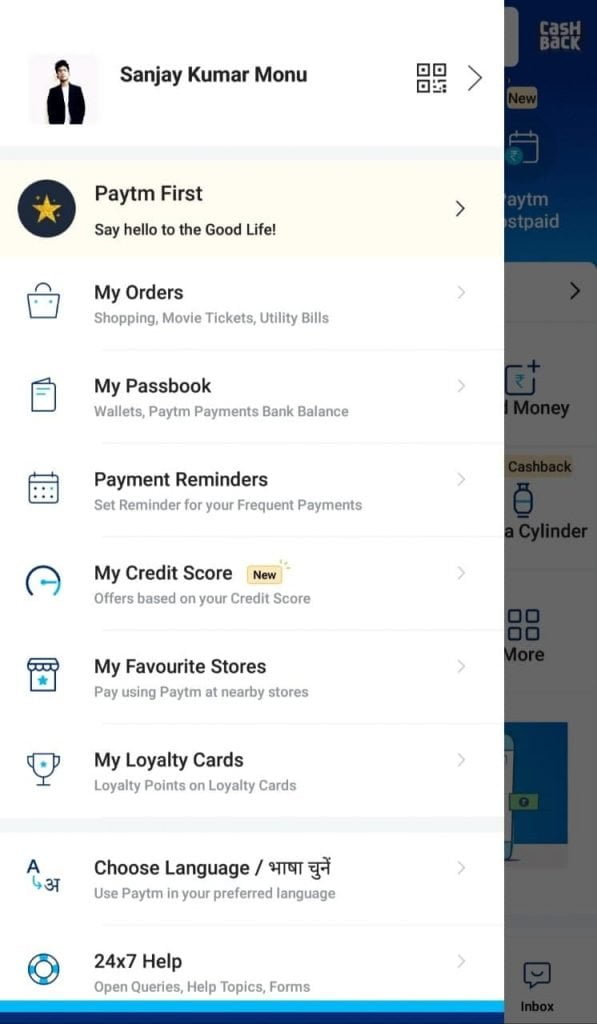Sure, here's a cleaned-up and detailed caption for the image:

---

The screenshot features a user profile of Sanjay Kumar Monu, dressed in a black blazer with a white shirt. At the top left corner is Sanjay's profile picture. The interface showcases four main sections, each represented by a shaded light pink rectangle with a black circle and star icon to the left, and a right-facing arrow to the right.

1. **PAYTM**: The first rectangle prominently displays "PAYTM" with the slogan "Say hello to the good life." This section likely serves as the main gateway for various Paytm services.
   
2. **My Orders**: The second section, labeled "My Orders," includes a shopping bag icon and options for managing shopping, movie tickets, and utility bills illustrated by a book icon.

3. **My Passbook & Wallets**: The third rectangle covers "My Passbook" and "Wallets," indicating services like Paytm Payments Bank Balance and Payment Reminders. A calendar icon suggests the feature to set reminders for frequent payments.

4. **My Credit Score**: The fourth and final section highlights "My Credit Score" with a red-orange rectangle labeled "New Offers Based on Your Credit Score." It includes a meter-like circular gauge with a stick, offering users insights related to their credit status and relevant offers.

Lastly, the interface hints at a feature called "My Favorite Stores," encouraging users to pay using Paytm at nearby stores, accompanied by an image of a typical store facade.